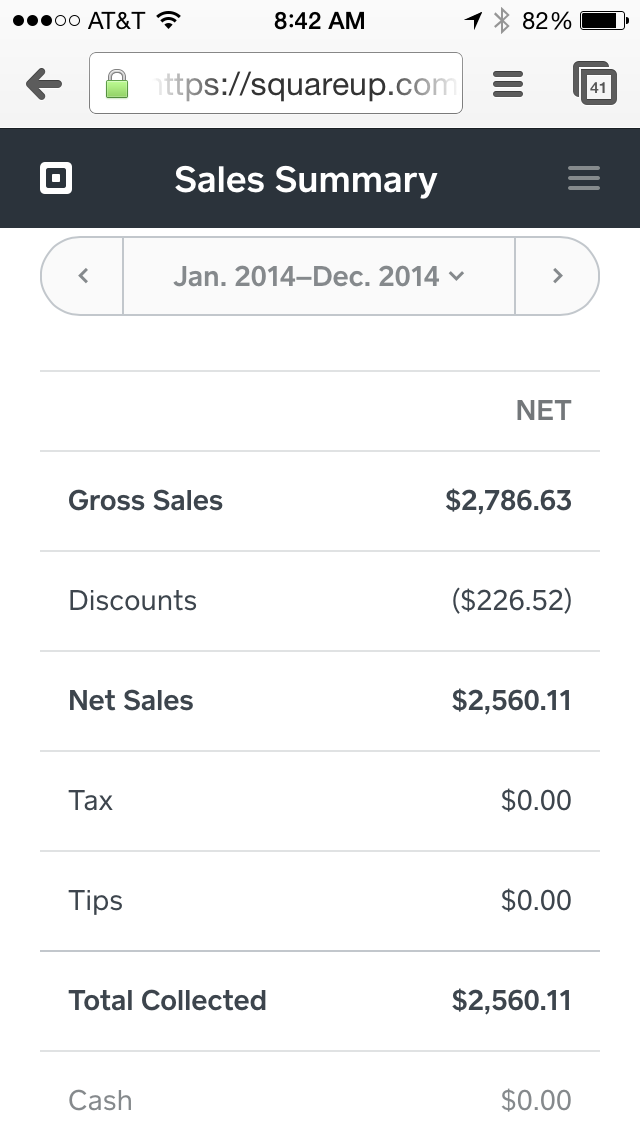The image is a detailed screenshot from a mobile phone showing a sales summary from a website. In the top left corner, it indicates the carrier AT&T with three out of five filled signal bars, and the time displayed is 8:42 a.m. The battery is at 82%, with a greyed-out Bluetooth symbol and an arrow symbol also visible. The website URL, "https://squareup.com," is partially greyed out. Below this, a blue header with white text reads "Sales Summary." The summary covers the period from January 2014 to December 2014. The gross sales amount to $2,786.63, with discounts totaling $226.52, resulting in net sales of $2,560.11. There are no taxes or tips applied, making the total collected exactly $2,560.11, and it shows no cash value.